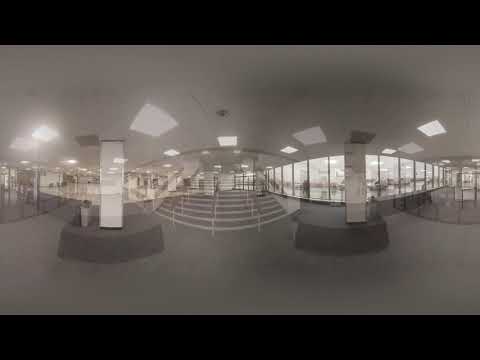This black and white photograph, framed with a thin black line on the top and a thicker one at the bottom, depicts a large and empty room, likely an exhibition space or a lobby in a shopping center. The room features a gray floor and a white ceiling equipped with a visible sprinkler system. Distorted slightly by the camera lens, the image shows two white pillars supporting the ceiling, creating an almost surreal geometric appearance with bent walls and hallways. A continuous row of large windows line one side, reflecting light from various sources across the ceiling. Although the image is grainy and overlaid with another hard-to-decipher image, faint outlines of people can be seen outside the window, adding an element of activity to the otherwise vacant and eerily lit space.